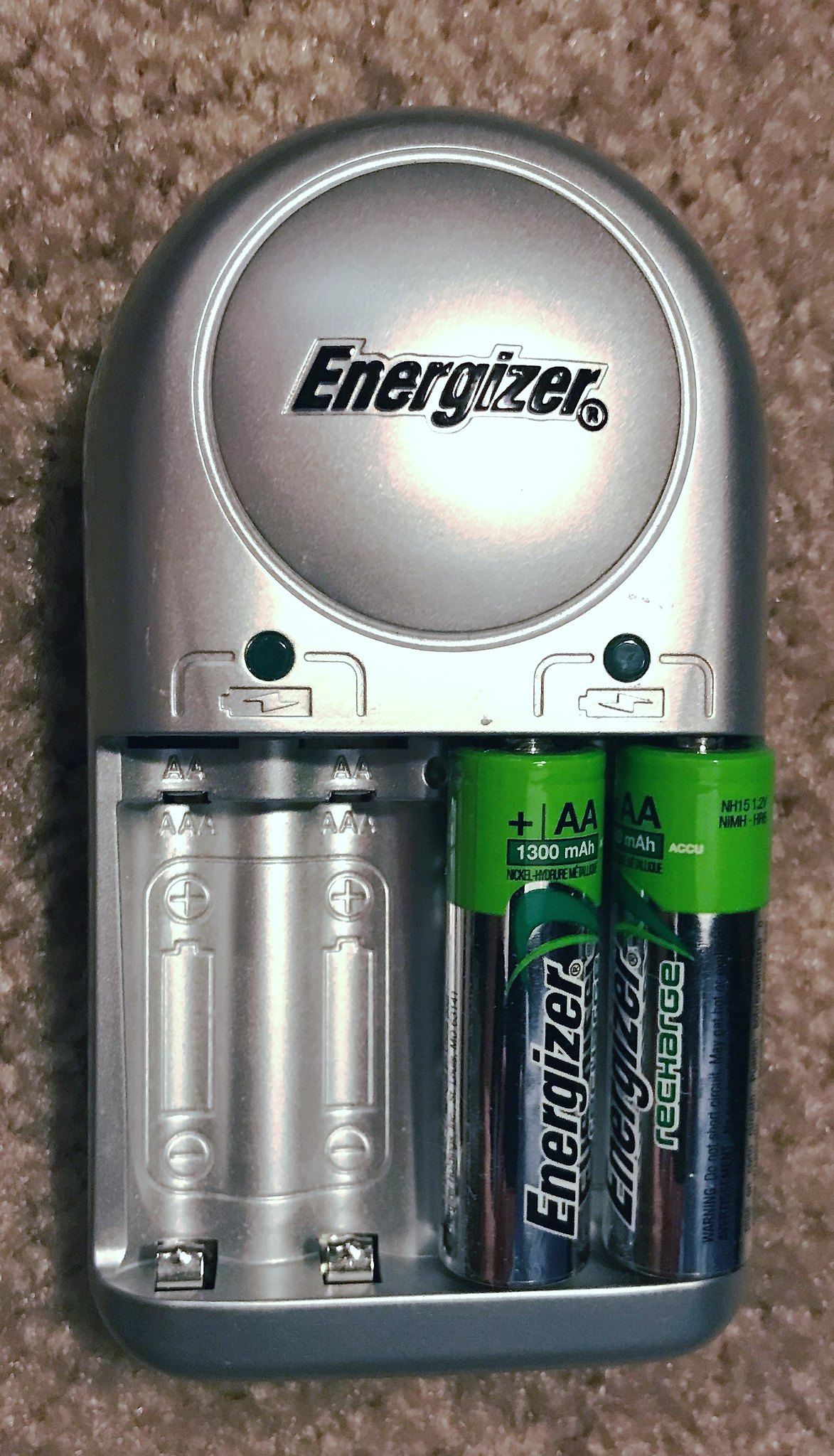This detailed image showcases an Energizer battery charger positioned on a carpet that resembles a brown oatmeal texture. The charger features a distinct design with a dome-shaped top transitioning into a rectangular base. The central part is silver-gray, engraved with the Energizer logo in black. It has a pair of green buttons, symmetrically placed on the left and right sides, with each side paired with a small indicator light. There are four battery slots: two are occupied by Energizer AA rechargeable batteries, distinguished by their green tops and silver bodies, marked with a 1300 mAh capacity, featuring a black Energizer logo with a white outline and a purple body. The other two slots remain empty. The device is unplugged in this setting, and additional details such as the small image of a battery on the charger, pointing left, are also visible.